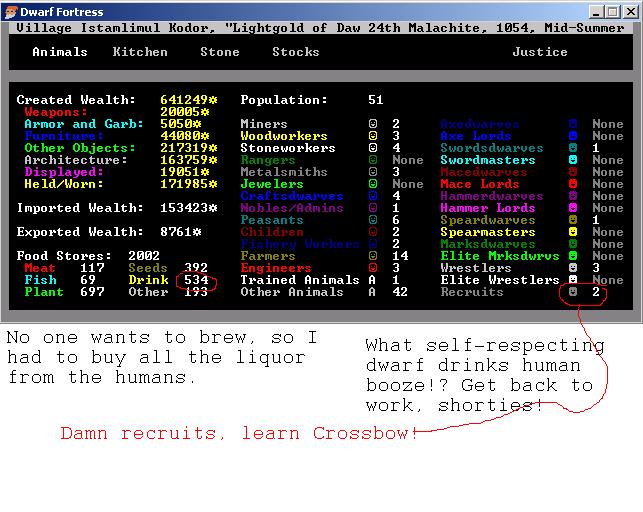This image is a detailed screenshot of an old game called Dwarf Fortress, evident from the title displayed on the blue bar at the top with the exit and minimize buttons. Below the title bar, the screen reads "Village Istamlimul Khodor, Light gold of Da 24th Malish Kite 1054 midsummer." The interface features several tabs, including animals, kitchens, stone, stocks, and justice, with the "animals" tab selected. Within that selection, it presents data such as created wealth (641,249), imported wealth (153,423), exported wealth (8,761), food stores (2,002), and population (51), categorized by different roles like miners, woodworkers, stoneworkers, and rangers.

Highlighted in red text and circled on the screen, there is a note that states, "Damn recruits learn crossbow" with a line pointing to an area marked "recruits." In a typewritten note outside the game screen text, it humorously reads: "No one wants to brew, so I had to buy all the liquor from the humans. What self-respecting dwarf drinks human booze? Get back to work, shorties!" The entire interface is typical of an old DOS-style program, showcasing a retro design aesthetic with colored text in shades of white, red, light blue, blue, green, purple, and gray.